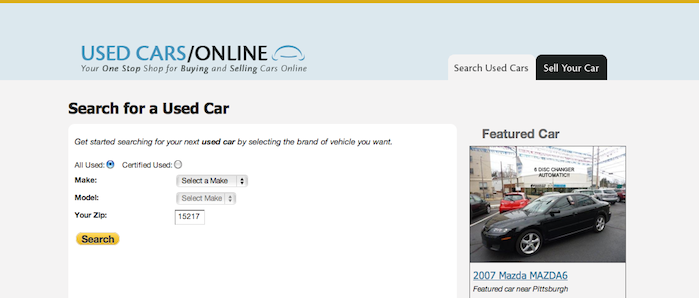The image is a screenshot of a website focused on buying and selling used cars online. At the top of the page, there is a prominent, thin yellow line. Below this line, a light blue border frames the main content area. On the left side of the blue border, the words "Used Cars / Online" are displayed in light blue against a black background, followed by the slogan "Your one-stop shop for buying and selling cars online."

To the right within this border, two tabs are visible: "Search Used Cars" and "Sell Your Car." The user appears to be on the "Search Used Cars" tab. The center section of the image, predominantly white, encourages users to start their search for a used car by selecting the brand of vehicle they want. The instructions are laid out in a clear format, with the words "Search for a used car" prominently displayed in black. Below this, there are fields to input the make, model, and zip code, followed by a yellow search button to submit the details.

On the right side of the screen, there is a section labeled "Featured Car," displaying an image of a black 2007 Mazda 6. The text beneath the image highlights that this is a featured vehicle near Pittsburgh.